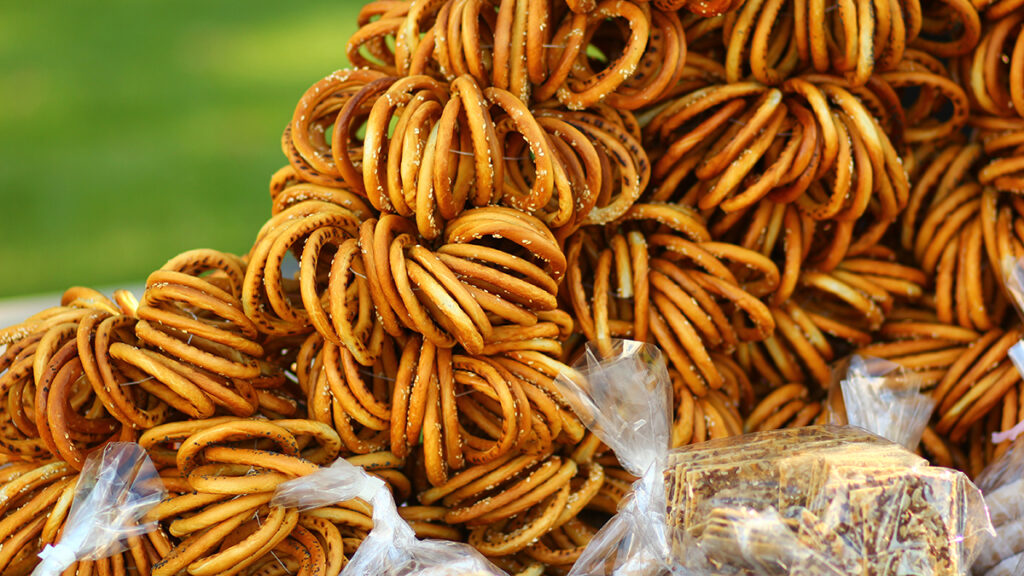This close-up outdoor photograph showcases a collection of brown, round objects resembling small pretzel rounds, each about an inch in diameter. Many of these pretzels bear white specks of salt, emphasizing their appetizing texture. They are mostly unbroken, though a few fragments are visible. The pretzels are notably arranged in groups, seemingly tied together in the center to form larger circular clusters, and they are partially nestled atop a plastic material. Towards the lower sections of the image, small plastic bags are interspersed among the pretzels, adding visual variety. The backdrop of the scene features a blurred expanse of green, likely grass, suggesting that the setting is an outdoor event, possibly a picnic or market table.